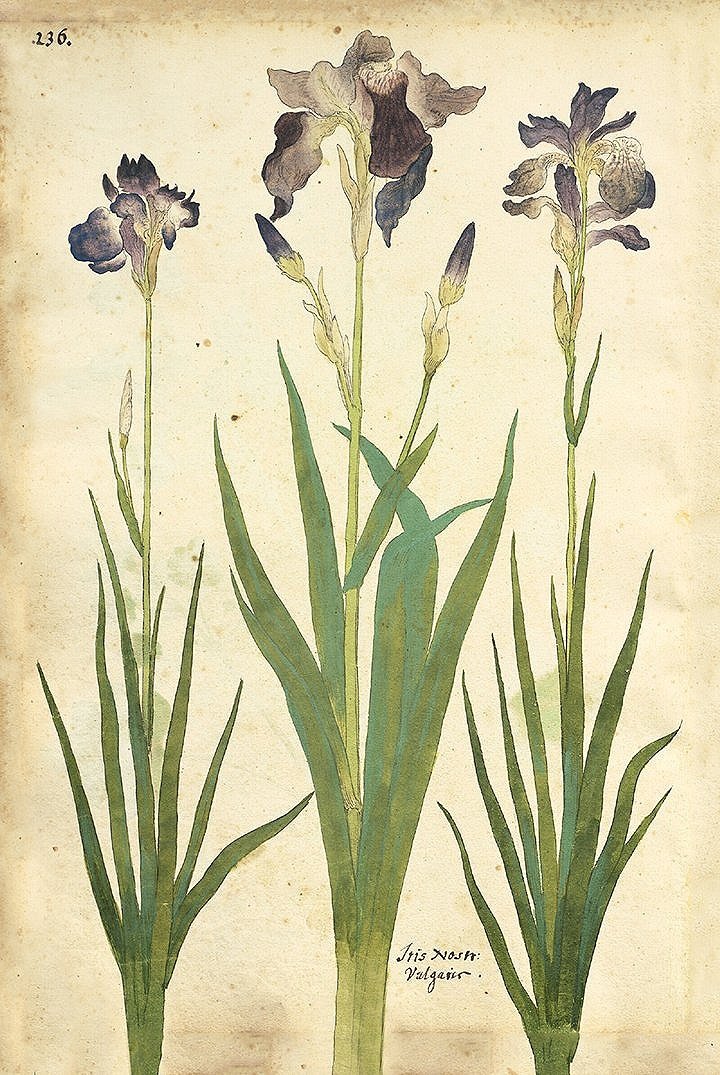The image features a detailed, aged botanical illustration on distressed, yellowing paper with a faded brown background, possibly resembling old parchment. The illustration depicts three tall, somewhat wilted irises with rippled purple and white petals. These irises have slender green stems and long, spiky leaves, some of which are bent. The largest iris is in the center, accompanied by two smaller ones on either side, each bearing buds. In the top left corner, the paper bears the tiny printed number "236" in a calligraphy font. Near the middle flower are words that appear to read "Iris Nostra," possibly followed by additional indistinct letters beginning with "B-O-L-G-E-I-R." This detailed botanical artwork combines the muted hues of green, purple, and brown, evoking a sense of antiquity and delicate beauty.